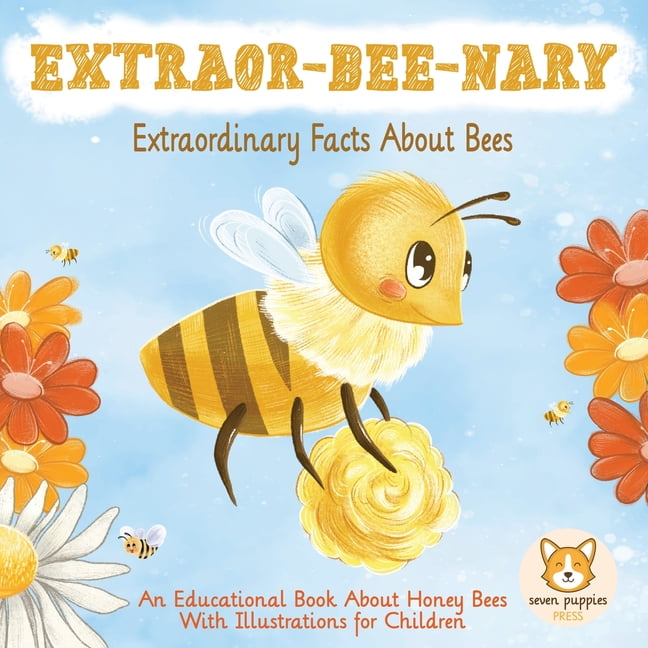The cover of this children's educational book is set against a light blue, sky-like background. Dominating the top of the cover is the creatively stylized title "Extraor-Bee-Nary," with a fun play on words that emphasizes the theme of bees. Just beneath this, in reddish lettering, the subtitle reads "Extraordinary Facts About Bees," clearly indicating the book's informative nature.

Central to the design is a charming, cartoonish bee with a large yellow head. It has human-like features, including big eyes and a friendly smile, along with black antennas and small white wings. The bee sports rosy cheeks and is surrounded by three smaller bees, adding a playful element to the illustration. Beneath the bee and slightly to the sides, colorful flowers in shades of white, orange, red, and yellow adorn the scene, enhancing the vibrant and cheerful aesthetic.

Positioned at the bottom of the cover, in red letters, is the description, "An educational book about honeybees with illustrations for children." To the bottom right, there is a light red circular logo featuring a smiling fox, accompanied by the name "Seven Puppies Press." Overall, the cover combines whimsical art and bright colors to attract and delight young readers while promising a wealth of fascinating bee facts.